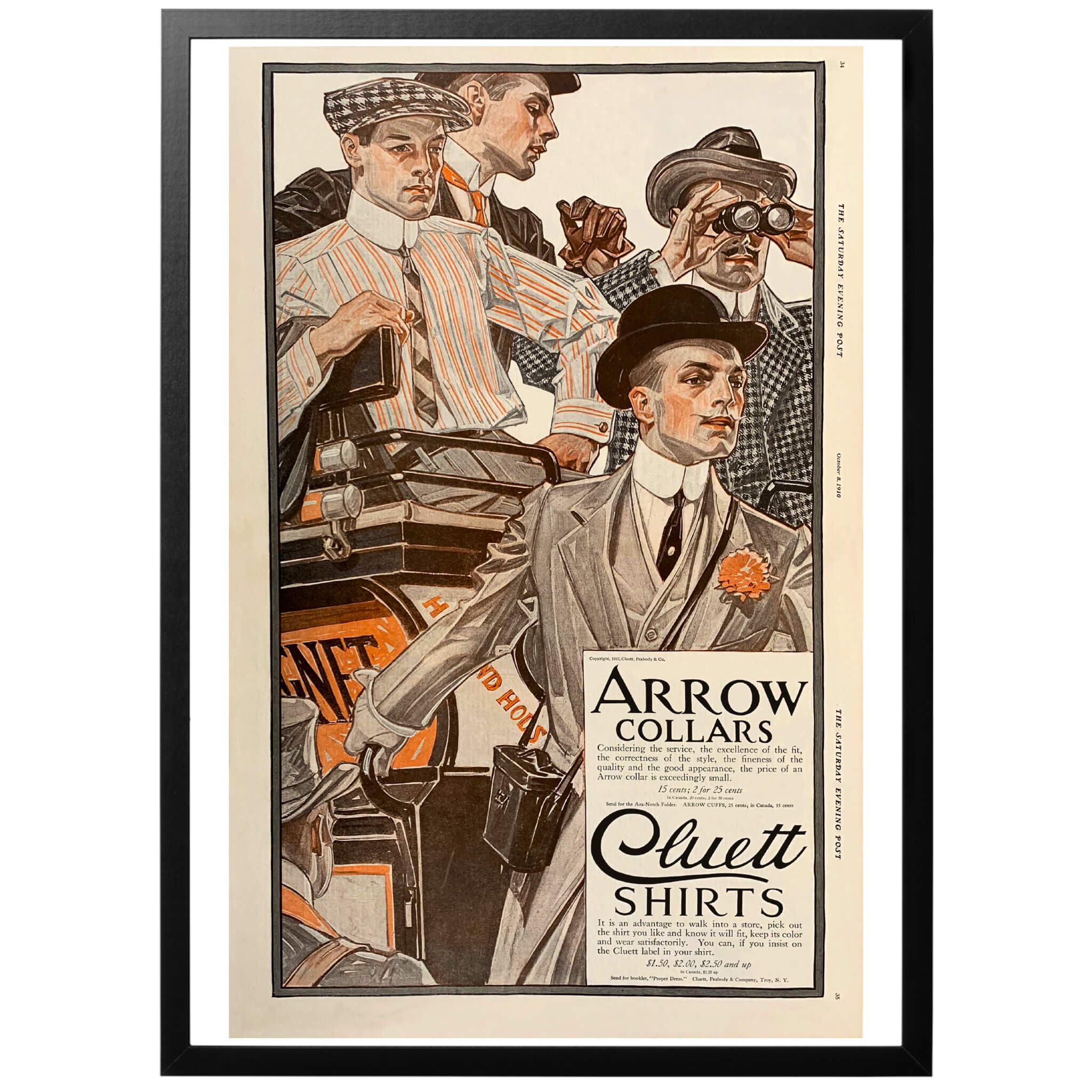The image is a framed, vintage advertisement for men's shirts featuring four men illustrated in various hats and outfits, each engaged in different activities. The frame is black, and the poster is on beige paper with its own black border. One man is holding binoculars, and another on the left is wearing a brown glove. The man in the front sports a bowler hat. At the bottom right corner of the poster, there is a caption in white with black lettering that reads "Arrow Collars" and "Cluett Shirts," followed by pricing details of $1.30, $2.10, and $2.50. Additional text beneath this indicates further information about Cluett shirts, although it is not fully legible. Along the right edge, the poster is marked with the words "January" and "The Evening Post," indicating its publication source.